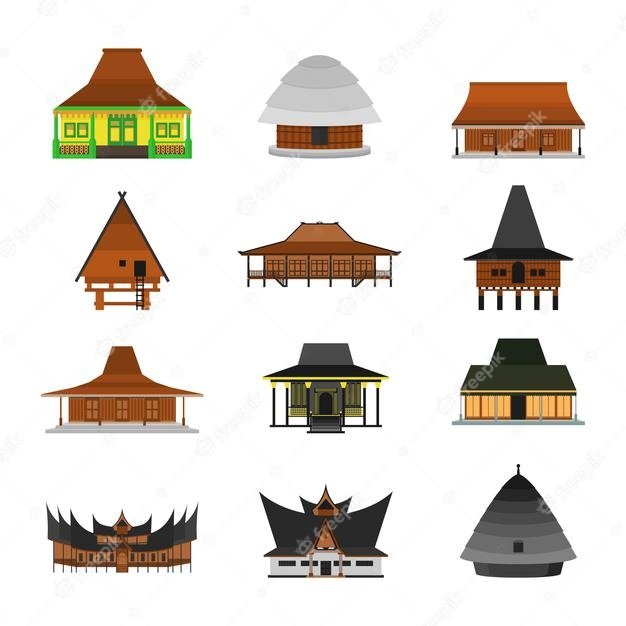The digital art image showcases twelve distinct and stylized building designs, arranged in a grid format with three rows of four buildings each, set against a white background. These buildings, which appear to represent various architectural styles not commonly seen in America, feature vivid color details and unique roof structures. 

In the first row, the top-left building resembles Mexican architecture with yellow siding, green wooden accents, and a blue, volcano-like roof. Adjacent to it is a building with an igloo-shaped top and a brown body. To the right, there's a structure reminiscent of a western-style house in brown.

The second row includes a teepee-shaped building, followed by one with Asian influences and another that features a roof resembling a witch's hat. 

The third row continues the Asian inspiration with buildings characterized by black color schemes with yellow detailing. This row includes a distinctive Asian-styled building with a black, layered roof.

The final row presents more Asian-inspired designs, including one resembling a spiky-roofed temple, another with a similar spiky roof, and a black building with a beehive-like top.

The overall image clarity is bright and clear, emphasizing the various shades of brown, black, gray, yellow, and beige used. The unique architectural designs, some with steep or layered roofs, and the consistent style and lighting, all contribute to this detailed, visually engaging image. A watermark stating "freepik" is also present across the image.